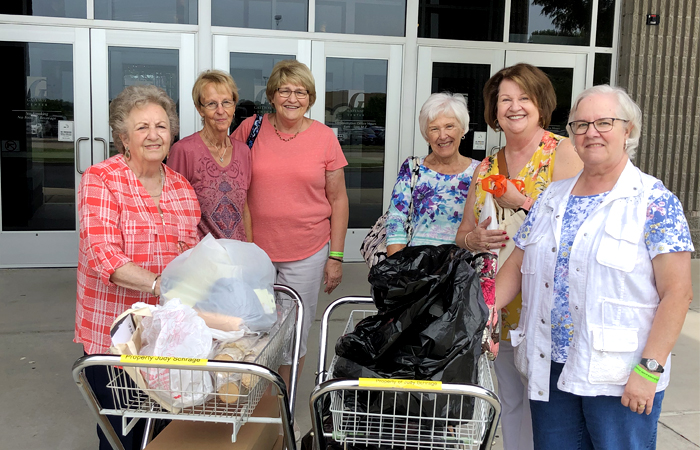In this photograph, six women, all appearing to be between their forties and seventies and likely above middle age, pose cheerfully in front of a building with glass doors that could either be a grocery store or a hospital. They range in hair colors from white to various shades of brown, and some have white hair. Their outfits are diverse, including red and white plaid tops, a solid salmon-colored top, floral prints, and one woman wearing a white vest. The women are gathered around two baskets – one on the left containing three to two white plastic shopping bags, and another on the right holding what looks like a black trash bag. The contents of these bags are not visible. The scene suggests an activity involving some sort of collaboration or mutual support, as all women stand close together, smiling warmly at the camera.